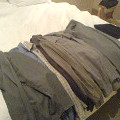In this very small, stamp-sized image, a pile of clothing, likely shorts, appears to be neatly laid out on what looks like a thick, gushy white blanket or bed sheet, heavily creased at the top. Multiple pairs of shorts in various colors are stacked on top of each other, arranged in what seems to be three separate piles. The leftmost short is black or very dark gray, the top right one is steel gray, and a pair underneath appears brown. The setting is probably a bedroom or household, though no other elements like pillows are visible due to the closely-cropped shot. Overall, the image captures the organized display of these vividly colored clothing items against the pristine white fabric background.